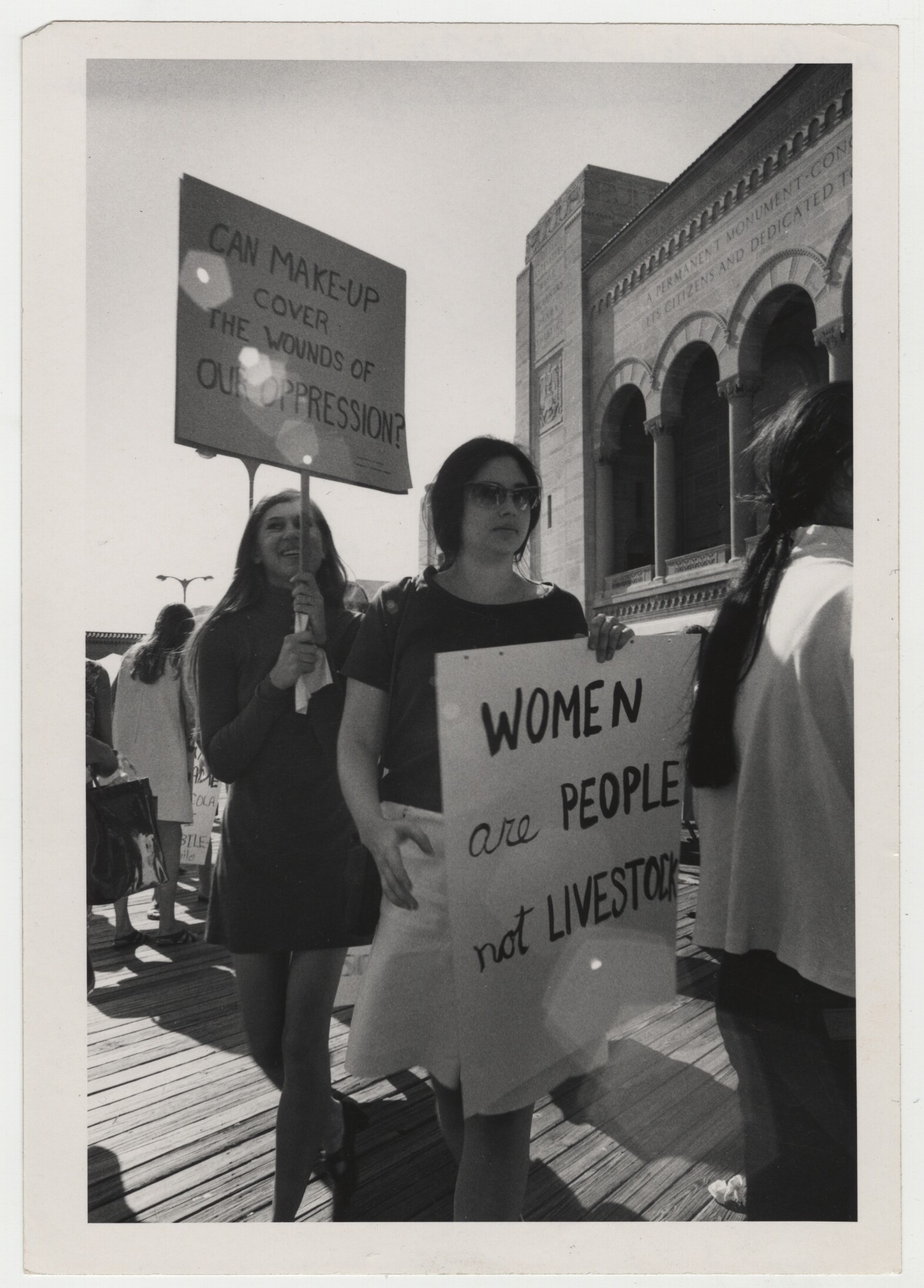The black and white photograph, framed by a thin white border with slight damage at the top left corner, captures a vibrant scene of a women's protest unfolding on a wooden boardwalk, possibly outside a pavilion. The setting features a striking building in the background adorned with Roman-style pillars and arches, suggesting an architectural influence from a foreign country, distinct from typical American design. The structure has inscriptions, but they are partially obscured: "the permanent monument" and "it's citizens and dedicated to," with the remaining text cut off.

In the center of the image, a woman with dark hair pulled back and wearing sunglasses stands resolutely, holding a sign in her left hand that declares, "Women are people, not livestock." Her outfit consists of a dark short-sleeved top and a white skirt. To her left, another protester, smiling and engaged, clutches a homemade wooden sign on a stick that reads, "Can makeup cover the wounds of our oppression?" She is dressed in a short, dark-colored dress. In the foreground, to the far right, partially out of frame, another individual with long dark hair tied in a ponytail is visible, wearing a white blouse and dark pants. Onlookers appear to be watching the demonstration, amplifying the scene's dynamism and sense of urgency.